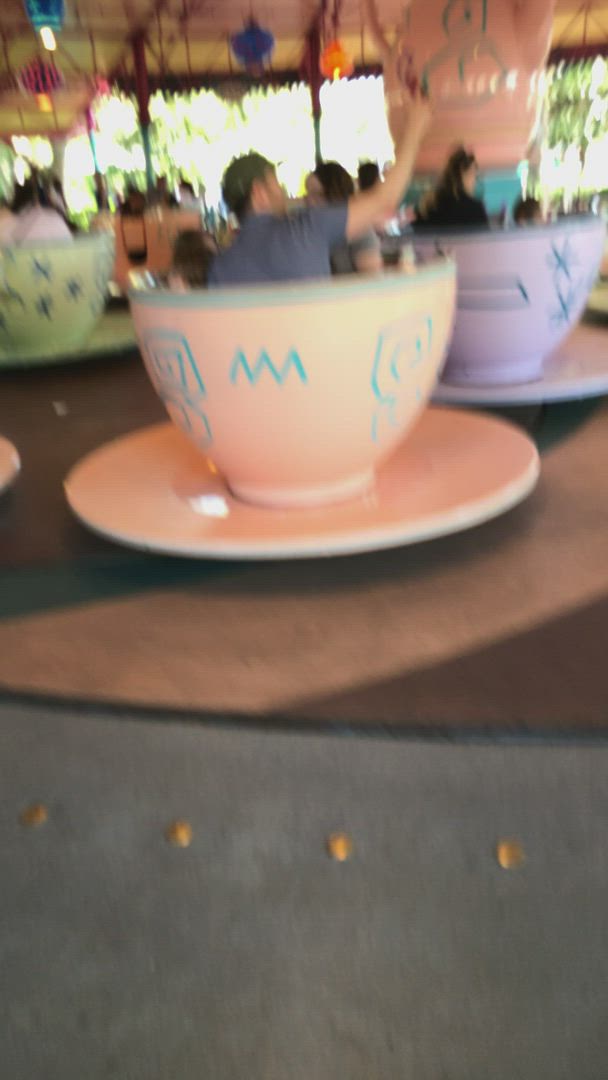A blurry image captures a vibrant, patterned teacup ride reminiscent of Disney World's famous attraction, but with a distinct cultural twist. The teacups, adorned with intricate etchings, give off an Asian or Egyptian aesthetic. In the foreground, a pale peachy-pink teacup with blue markings hosts a man in a blue shirt, who appears to be either waving or taking a picture. To the left, a lime green teacup and to the right, a purple teacup, both similarly decorated, each with riders enjoying the spin. In the background, blurred figures wait in line under a canopy adorned with what seem to be Japanese lanterns. Greenery peeks through the structure, adding a touch of nature to the scene, though the image remains notably indistinct.